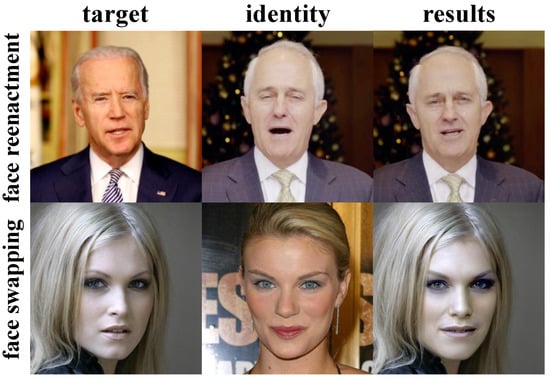The illustration depicts a grid of six edited photos, arranged in three columns and two rows, showcasing face merging and reenactment techniques. The left column, labeled "Target," features a top image of Joe Biden in a suit and a bottom image of a young blonde woman. The middle column, labeled "Identity," includes an older man in a suit resembling Biden and another blonde woman whose expression is slightly altered compared to the "Target" image. The right column, labeled "Results," presents the results of combining the corresponding "Target" and "Identity" faces, with the top row showing an elderly man merging with Biden's features and the bottom row showing a blonde woman with a subtle expression change. The top row is titled "Face Reenactment," and the bottom row is titled "Face Swapping." The color scheme includes shades of gray, white, blue, black, and hints of yellow. This image is likely a demonstration of face-melding technology using political and neutral figures.